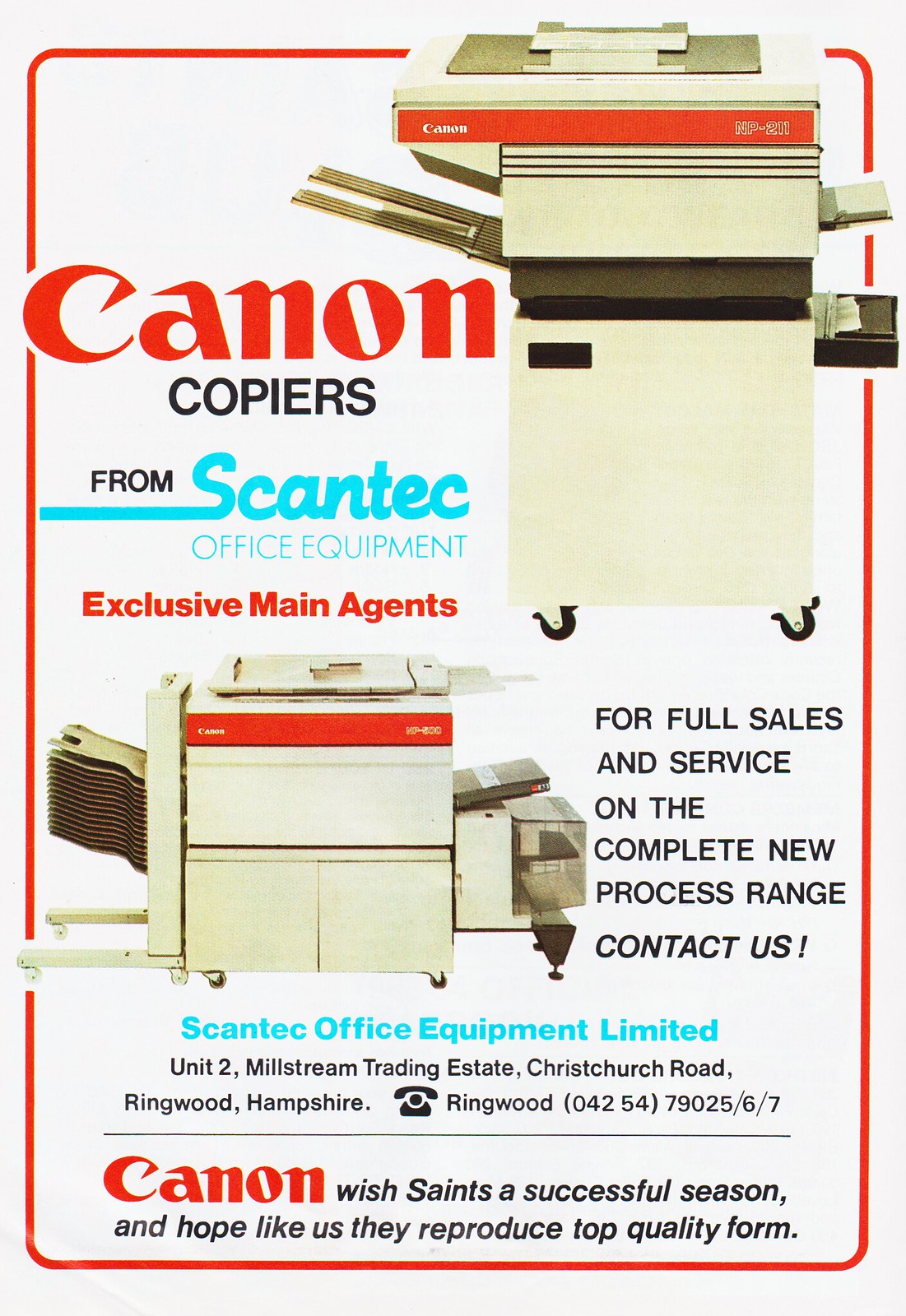This vertically aligned rectangular advertisement features a bold red border surrounding a white background. In the upper portion, the poster prominently displays a large, high-quality image of a Canyon copier machine on the top right. Adjacent to the copier image, in large red letters, it reads "CANON"; beneath this, "COPIERS" appears in black. Below these texts, the phrase "FROM SCANTECH OFFICE EQUIPMENT" is highlighted in blue, followed by "EXCLUSIVE MAIN AGENTS" in red. 

Further down, two images of different-sized Canon copiers are displayed: one situated on the middle left and another, larger machine, towards the bottom center. To the right of the larger copier image, the statement "FOR FULL SALES AND SERVICE ON THE COMPLETE NEW PROCESS RANGE CONTACT US" is displayed in black. Below this message, in blue letters, it reads "SCANTECH OFFICE EQUIPMENT LIMITED", followed by the address "Unit 2 Millstream Trading Estate, Christchurch Road, Ringwood, Hampshire" and the phone number "(04254) 79025/6/7" shown in black.

At the very bottom, the text concludes with "CANON" in red letters once more and the supportive message "WISH SAINTS A SUCCESSFUL SEASON AND HOPE LIKE US, THEY REPRODUCE TOP QUALITY FORM" in black. The overall layout, punctuated by a thin blue line and detailed imagery, effectively showcases the featured Canon copiers and highlights Scantech Office Equipment Limited's exclusive agency and contact information.